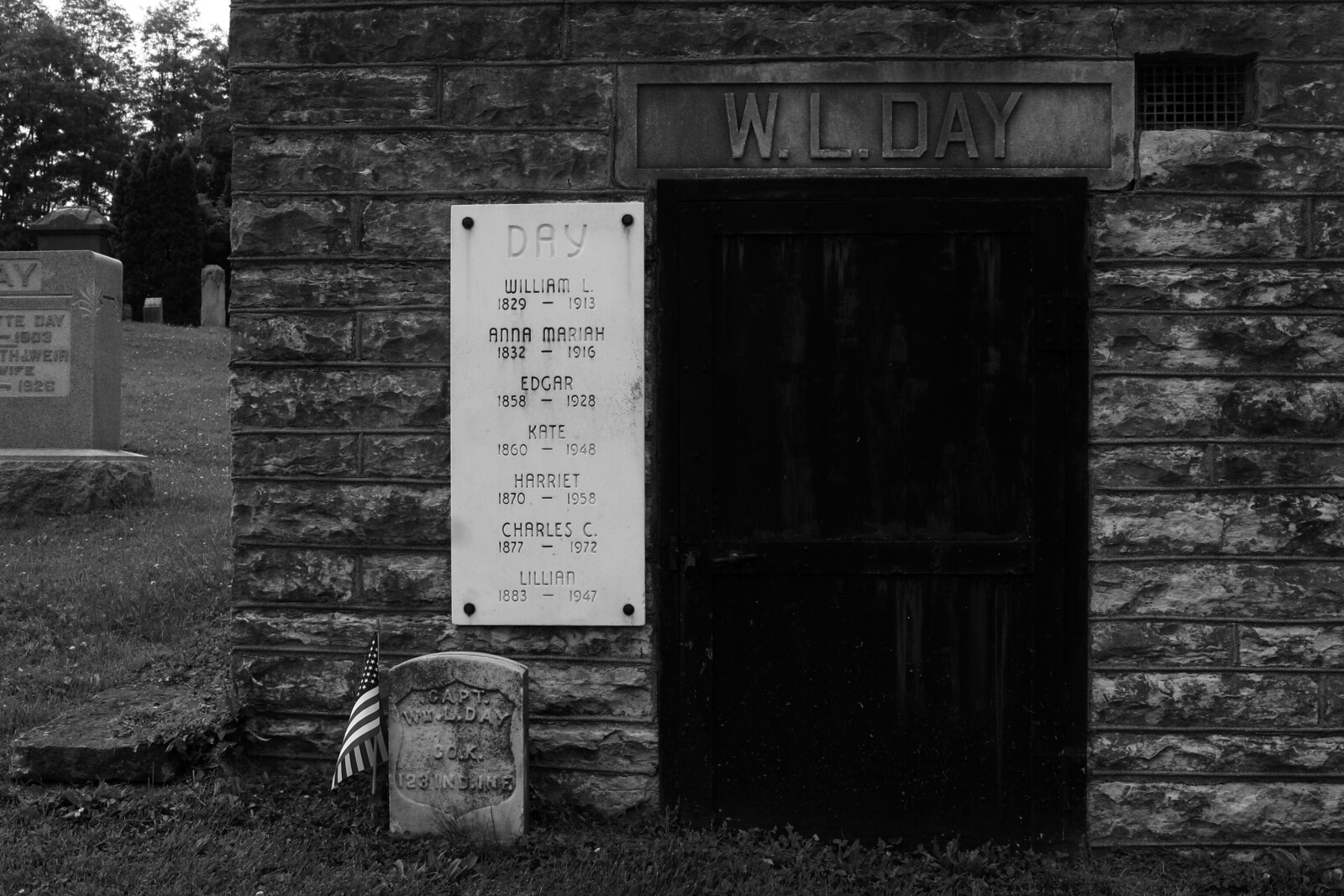In this detailed black-and-white photograph of a graveyard, gravestones can be seen off to the far left side, partially embedded in what appears to be a grassy hill. Dominating the picture, from nearly the left edge to the right edge, is a large stone crypt made of gray and black bricks, bound with flat mortar. This crypt features a prominent doorway with a large, dark brown wooden door. Above the doorway, etched in stone, are the initials "W.L. Day." To the left of the doorway is a white rectangular plaque that lists the names and lifespans of several individuals: "Day," followed by "William L. 1829-1913," "Anna Maria 1832-1916," "Edgar 1858-1928," "Kate 1860-1948," "Harriet 1870-1958," "Charles C. 1877-1972," and "Lillian 1883-1947." In front of the crypt, near the plaque, is a tombstone accompanied by an American flag planted beside it. In the background, beyond the crypt, the sky is a stark white, which contrasts with the silhouettes of trees.